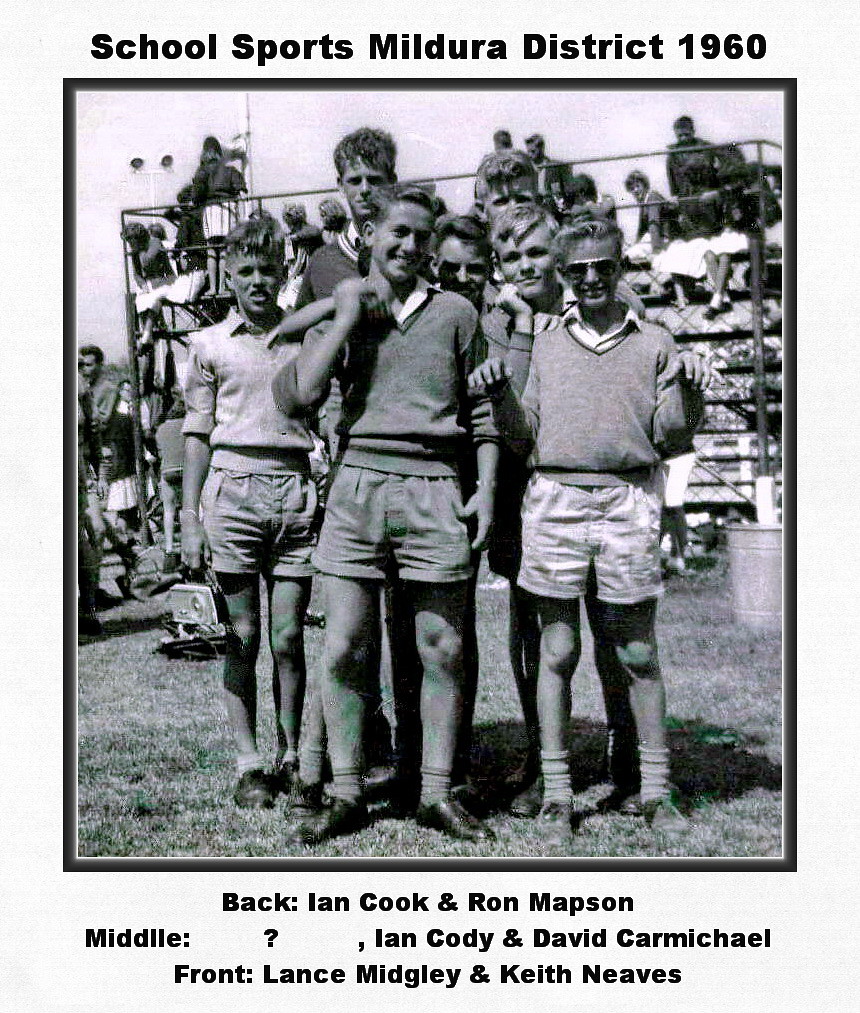In the center of the image, a vintage black and white photo from the 1960s captures a group of young men posing on a grassy field. The photo is bordered in black, and at the top, bold black text reads, "School Sports, Mildura District, 1960." At the bottom, in centered black lettering, it identifies the individuals: "Back: Ian Cook and Ron Mappson. Middle: ?, Ian Cody, and David Carmichael. Front: Lance Midgley and Keith Neves." The group, consisting of two individuals in the front, three in the middle, and two in the back, is dressed in shorts, jumpers, and polo shirts. One person on the right wears sunglasses. Behind them, you can see bleachers filled with children, some facing forward, others looking backward, and a few kids walking on the grass to the side. The young men in the photo are smiling and facing the camera, showcasing the casual and cheerful atmosphere of the school sports event.